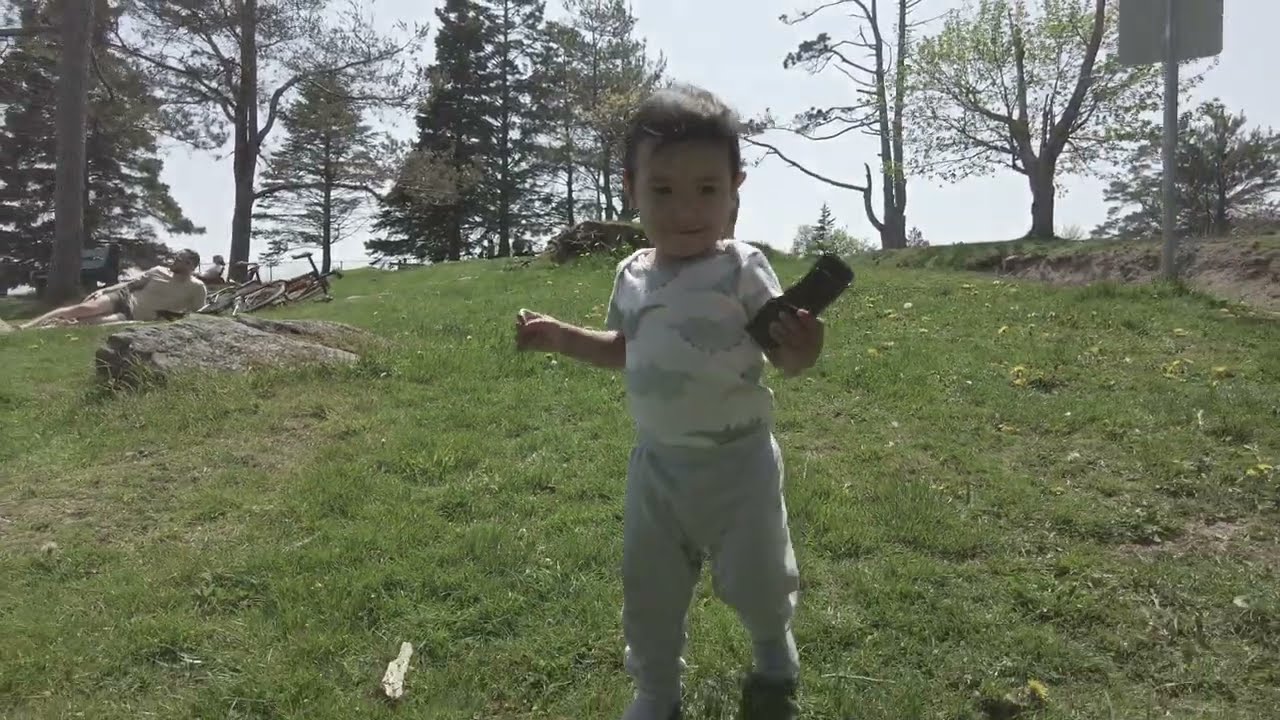In a color landscape photograph, a young toddler, around two years old, stands at the center in a grassy, hilly park area. The child, with dark short hair and dark skin, is wearing a white shirt with gray patterns and gray sweatpants. He appears to be holding a dark object, possibly a cell phone, in his left hand while his right hand remains empty. He gazes downward, focusing on his steps, with a subtle smile on his face. The scene is bathed in natural light, casting gentle shadows as the sun is behind him, creating a slightly darker appearance on his figure. In the background, the park extends with lush grass, a scattering of trees, and a hazy sky that is predominantly whitish with hints of blue. To the child's right, a man in a yellow t-shirt and greenish shorts reclines on the grass, looking away into the distance. There is a sign on a pole on the right side of the image, faced away from the viewer, and a couple of bicycles lie flat on the grass near a large rock. This photographic representation captures a serene, everyday moment in a park setting, emphasizing the tranquility and exploratory nature of the child's surroundings.